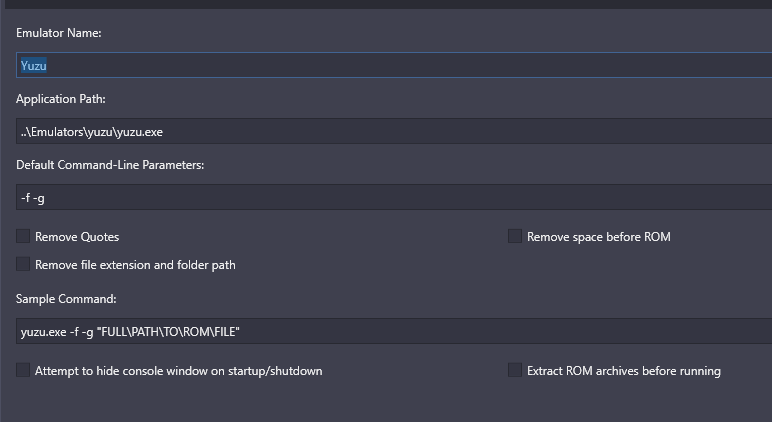**Detailed Caption:**

A screenshot from a website interface displaying configuration settings for the YUZU emulator. In the upper left corner, the title "Emulator Name" is depicted, paired with the name "YUZU" written in light blue font, which is enclosed within a darker blue highlight or box. This section is further outlined with a blue border.

Beneath it, a field labeled "Application Path" shows the directory navigation to the YUZU executable file: `\emulators\YUZU\YUZU.exe`. 

The next section is titled "Default Command-Line Parameters" which includes two parameters listed in the data field: `-f` and `-g`, both in lowercase. 

Options for "Remove Quotes" and "Remove File Extensions and Folder Path" are present with accompanying checkboxes, though neither checkbox is marked.

Further down, the label "Sample Command" is presented, and the corresponding data field contains the simulated command: `YUZU.exe -f -g "FUL\path\to\ROM\file"`.

Finally, an additional setting at the bottom mentions "Attempt to Hide Console Window on Startup and Shutdown" followed by a forward slash. The visual shows a clean and structured layout for configuring the YUZU emulator via this website interface.